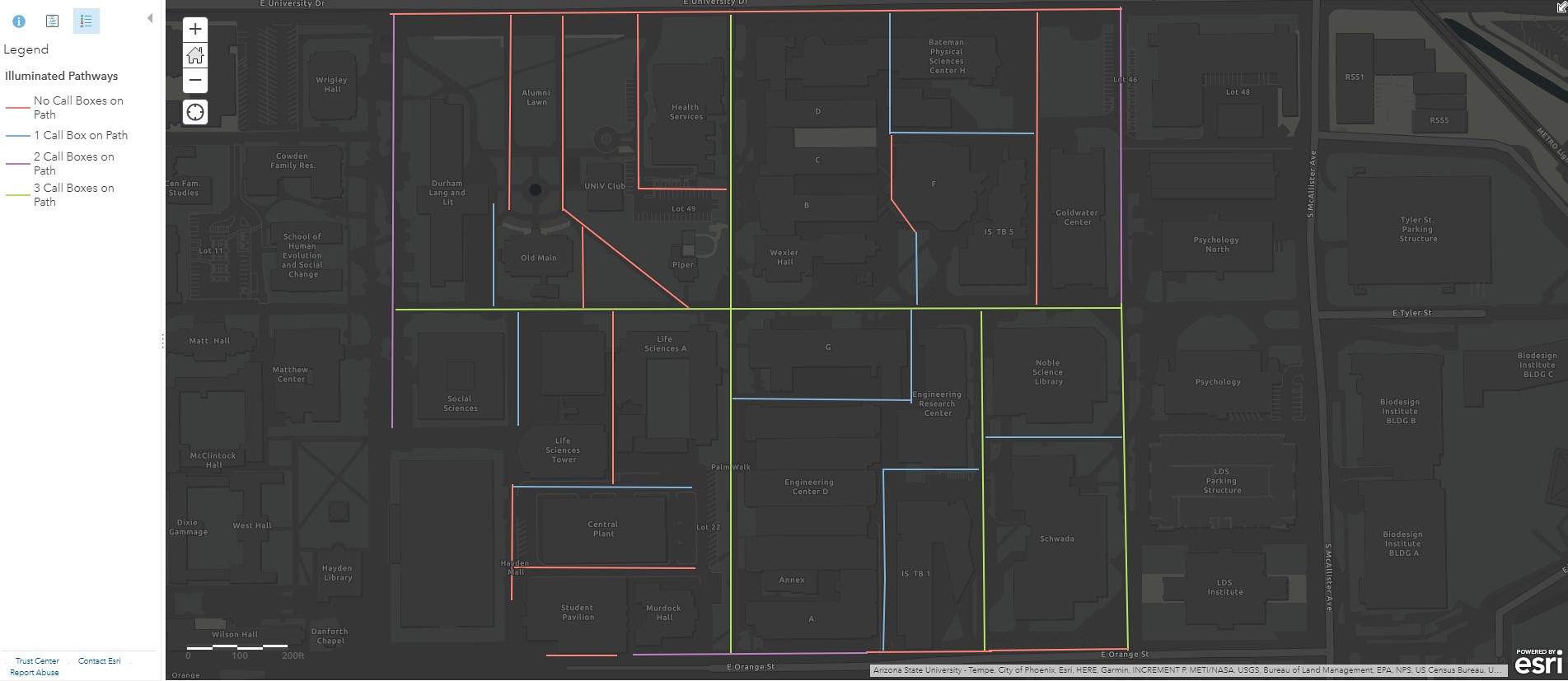The image displays a rectangular graphic with a stark black background, adorned with an array of lines in multiple colors: purple, red, yellow, and blue. These lines intersect and form various geometric shapes such as squares, rectangles, and triangles. On the left side of the graphic, a legend is present, labeled "Numerical Pathways," identifying each colored line. The red line, which is difficult to read but appears to be labeled "Callie" or something akin to it, is followed by a green line labeled "One cell." Further down, there is a purple line marked "Two cell," and a yellow line named "Three cell." Additionally, there is indecipherable text within the shapes created by these lines on the black background.